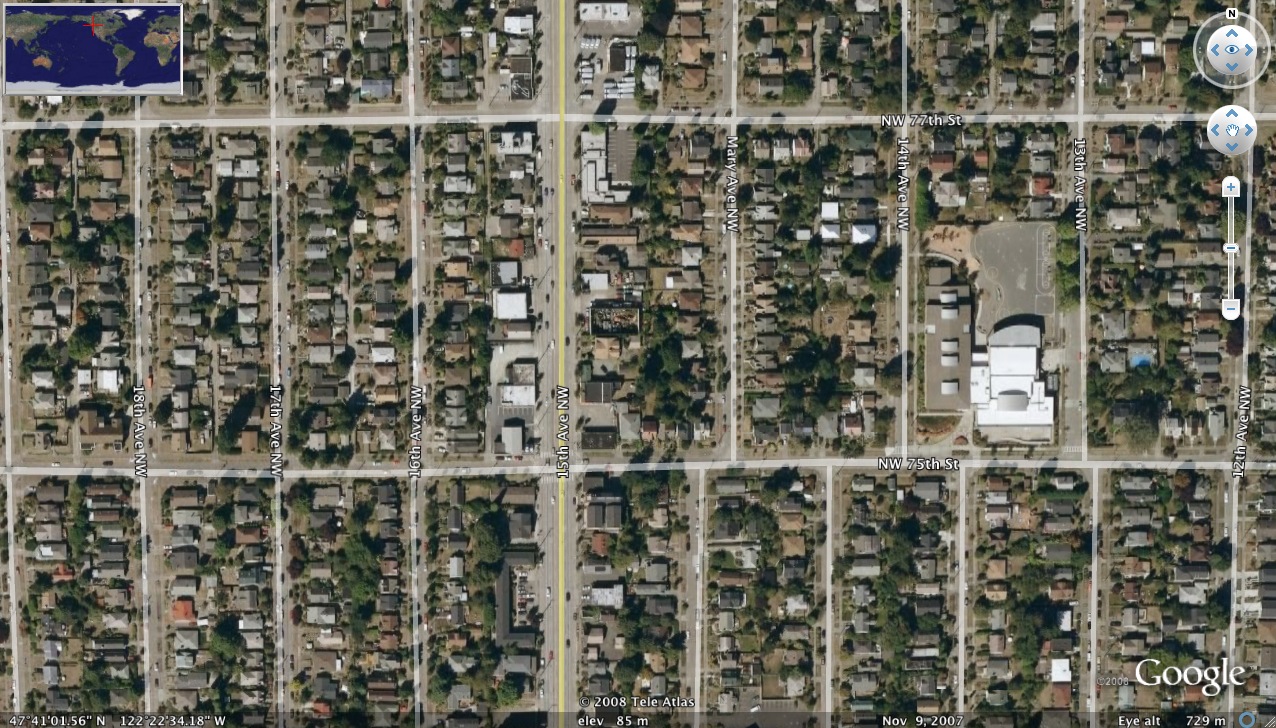This image is a detailed satellite screenshot from Google Earth, capturing a suburban neighborhood with a meticulously organized grid of streets. The aerial view clearly shows numerous buildings and clusters of houses laid out in rectangular patterns. Dominating the image is the central yellow-labeled 15th Avenue Northwest, surrounded by various other street names.

In the upper left corner, a small world map features a red orientation cross pinpointing the upper western United States, likely positioned over Washington or Oregon. The upper right corner displays a compass for directional reference, accompanied by a zoom slider below for adjusting the map's scale. Despite the absence of explicit labels indicating the specific city or town, the detailed street names provide a sense of the area's layout and structure.